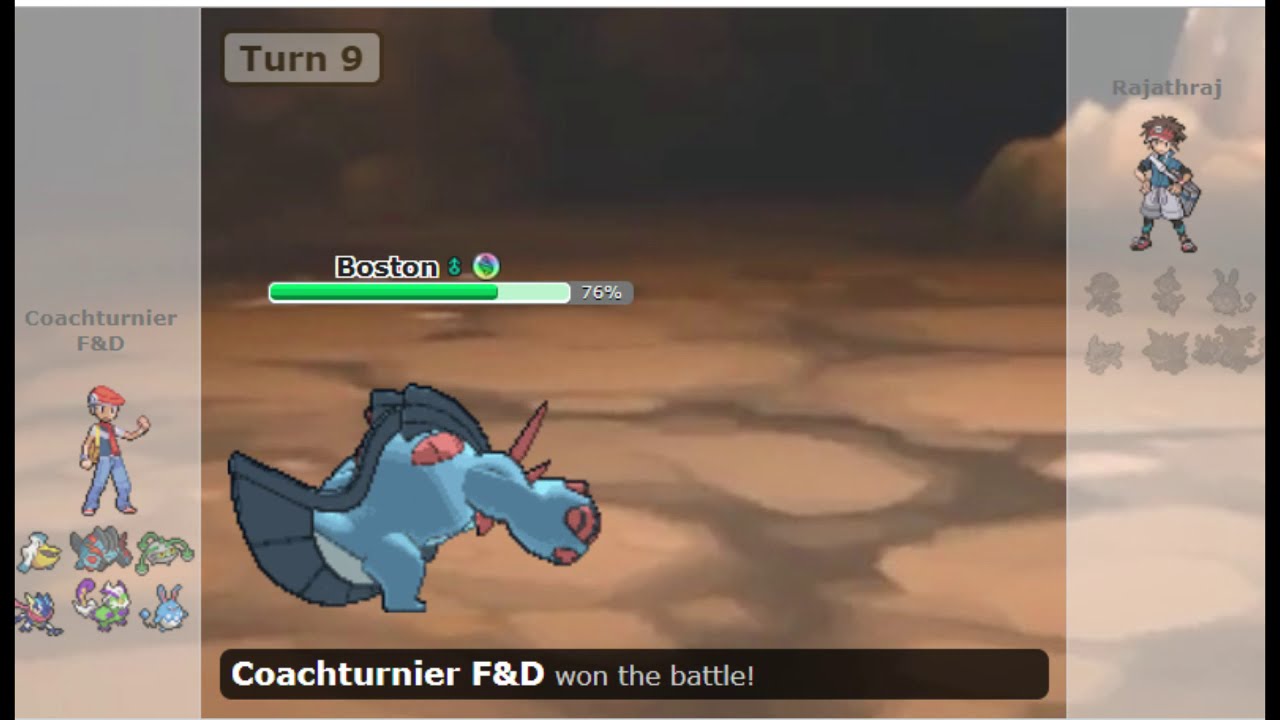The screenshot is from an old-school, pixelated video game that resembles a Pokémon-style battle scene. Dominating the center of the image is a blue, fish-like creature with dark blue wrappings and several red markings, including a red horn on its head, blotches on its back, and spots on its snout. This creature stands on a stone floor, presumably in a cave setting. Above the creature is a health bar labeled "Boston," showing 76% health. 

In the upper left corner, the word "Turn" followed by the number "9" is displayed. Below this, a green progress bar indicates the remaining health. The left side of the image features a vertical strip with a character—likely the coach—wearing a hat with red detailing and blue pants, holding one fist in the air. Beneath this character, there are six different options for creatures. Some of them include unique animals like a pelican, while others are less distinguishable.

On the right side, there is another character with an Indian headdress, a blue shirt, and grey shorts. Above this character, the names "Rajat, Ha, Raj" are shown. Below this character, the creature options are greyed out, indicating they are likely unavailable for selection at this time.

At the very bottom of the image, white text on a black strip reads, "Coach Turnier F&D won the battle!" with an exclamation mark at the end, celebrating the victory in this turn-based battle game.